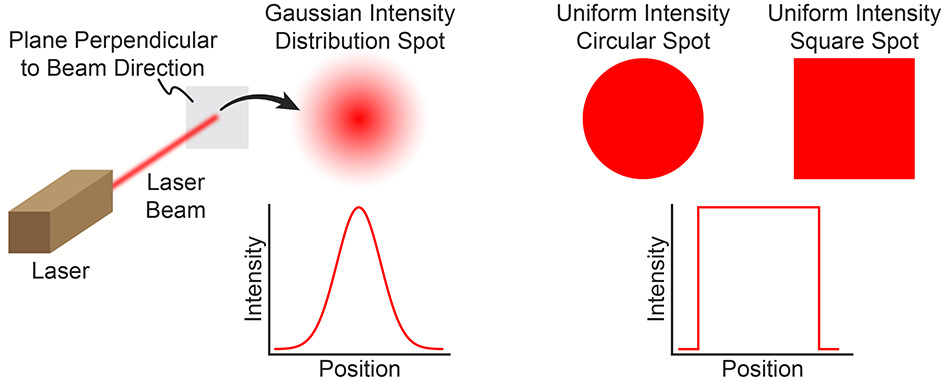The image is a detailed scientific diagram illustrating various laser beam intensity distributions. At the top left, there is the text "beam perpendicular to beam direction," accompanied by a depiction of a laser emitter firing a laser into a gray square. The gray square directs attention to different types of beam spots. First, an arrow points to a blurred red dot labeled "Gaussian Intensity Distribution Spot," which is characterized by a specific graph showing how intensity changes with position—narrowing at high intensity and broadening at lower intensity. To the right, there’s a focused red circle labeled "Uniform Intensity Circular Spot," and further right is a red square labeled "Uniform Intensity Square Spot." Below the main illustrations, there are two charts showing intensity versus position, with respective diagrams to further illustrate the data. All text and labels in the image are in black.